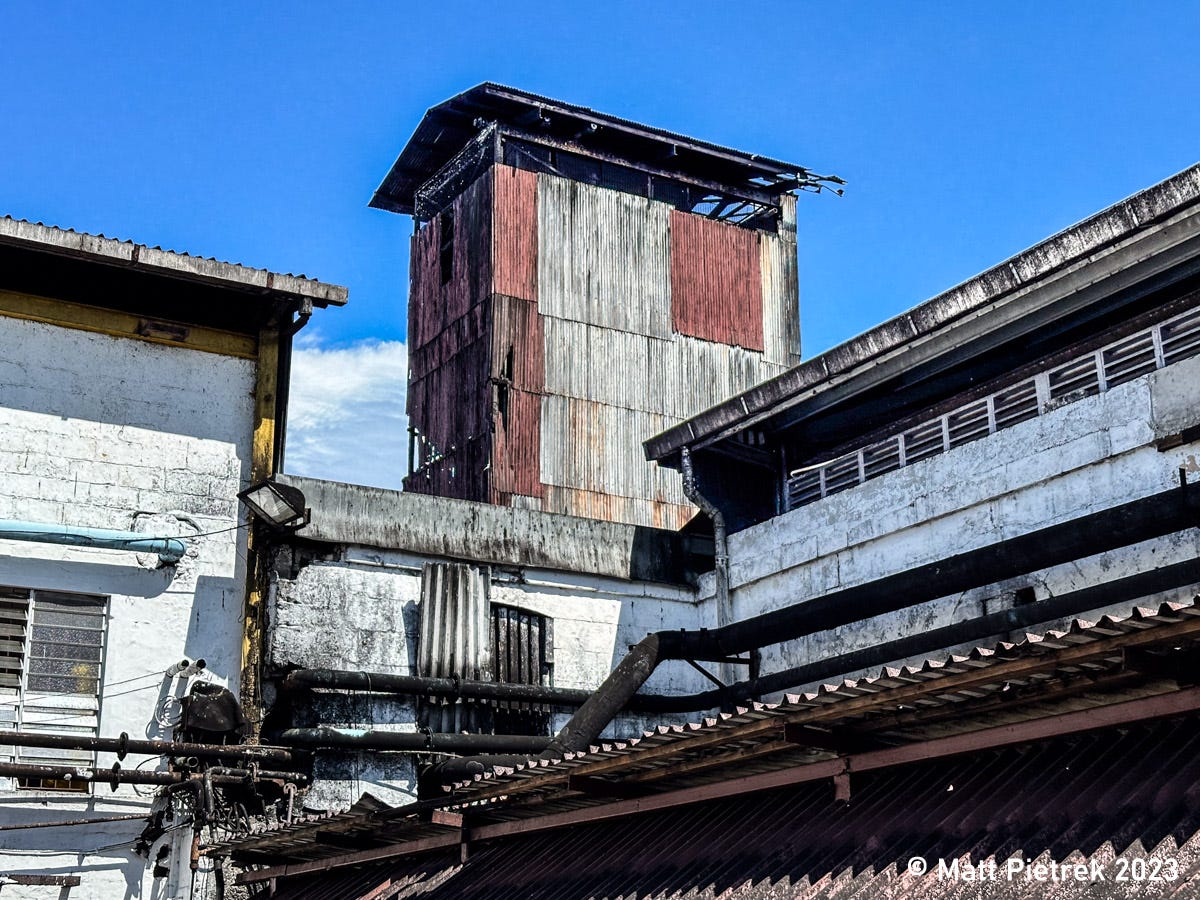The photograph, taken by Matt Pietryk in 2023, showcases an old, dilapidated industrial building under a beautiful, clear blue sky with a few scattered clouds near the horizon. The building, likely an abandoned factory or storage facility, features multiple add-ons and structures that speak to its age and state of decay. One prominent building in the background is covered with corrugated aluminum sheets, which are rusted and have holes where siding has fallen off. The roof of this building also shows signs of significant wear with visible gaps. Adjacent to this structure, there's a white building with brick sections patched up with tin and red sheet metal. The complex network of tubes and pipes running between the buildings adds to the industrial ambiance, while tin awnings remain as relics meant to manage rainwater. Overall, the imagery of decay and disrepair is set against the stark contrast of a serene blue sky, making the photograph both dramatic and evocative. In the bottom right corner, the image is credited with the text "© Matt Pietryk, 2023."